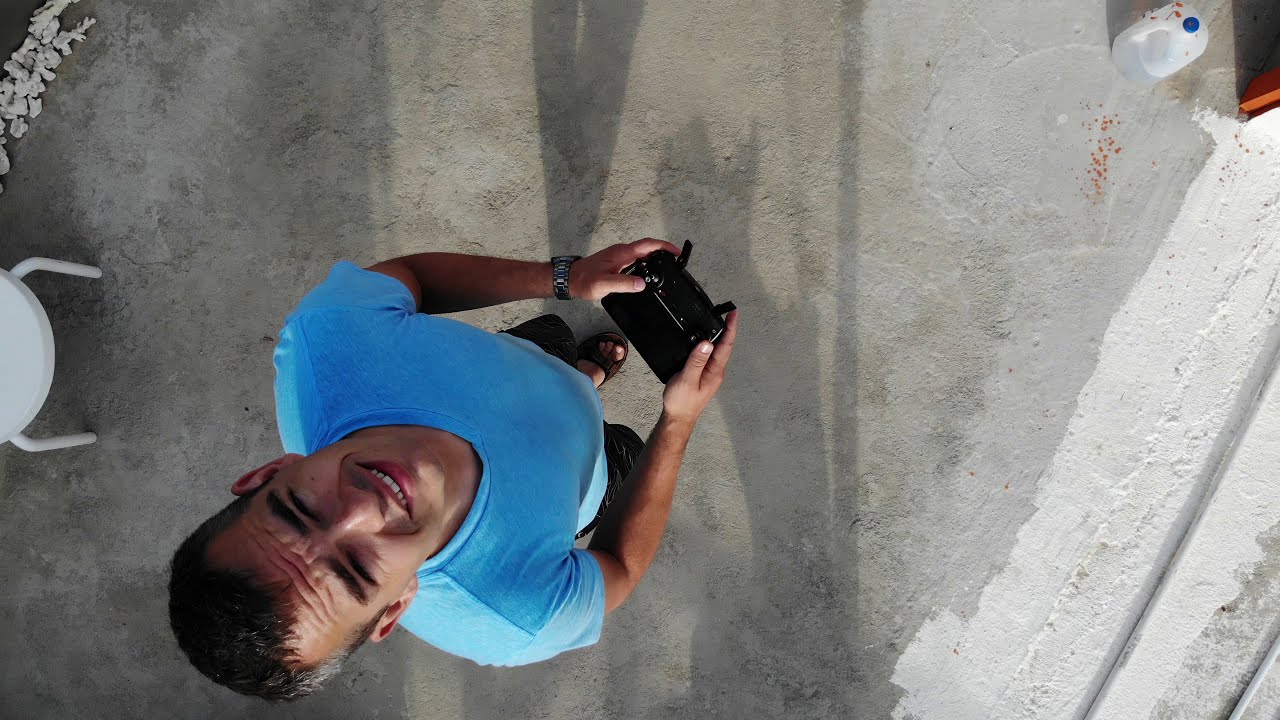The image is a drone photograph taken from directly above a man in his 20s or 30s, who is presumably taking a self-portrait. The drone seems to be hovering about 10 feet off the ground, as indicated by the clear visibility and detail of the man and his surroundings. The man is standing on a concrete or cement patio, which appears to be painted grey and white in some areas. He has short cropped black hair with a possible touch of grey, black eyebrows, olive or brown skin, and is wearing a blue t-shirt and black shorts. His footwear consists of open-toed sandals. He is holding a black rectangular controller, resembling a video game controller with two small antennae, in front of his body. He is looking almost straight upwards at the drone, squinting his eyes, likely due to the sunlight behind the drone. The photo also shows his shadow cast on the ground. To the left side of the image, there is a small, simple white patio table or stool with two legs that look like small pipes. In the upper right-hand corner of the photo, there is a gallon jug of water. The overall setting is a concrete patio with a few objects, focusing mainly on the man and his interaction with the drone.